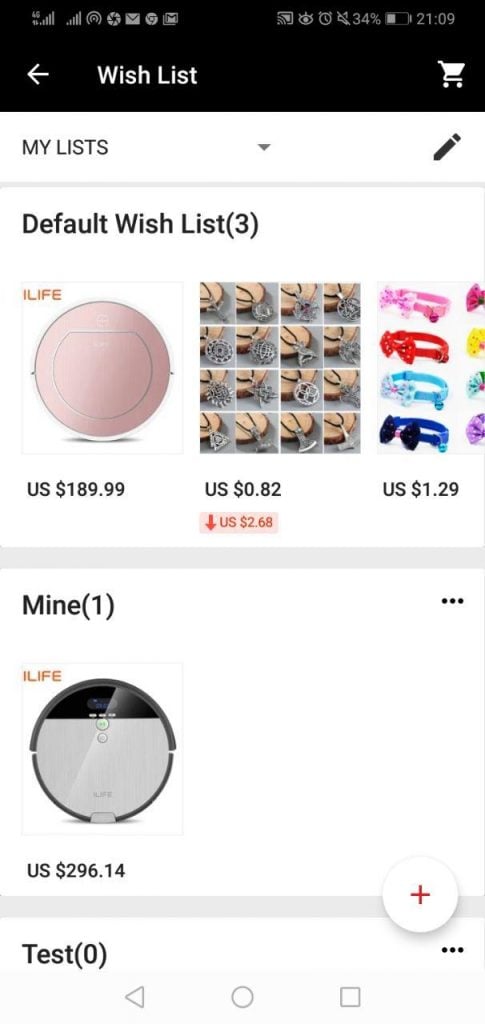The image is a screenshot from a mobile device displaying a detailed view of a wish list within a shopping app. Across the top, a black status bar is filled with small icons indicating various statuses such as signal strength, email, battery status, speaker, time, and more. Below the status bar, the app's navigation features a left-pointing arrow, the text "Wish List," and a shopping cart icon positioned on the far right.

The main section of the screen, set against a white background, begins with the title "My Lists" on the left side. Adjacent to this title is a universal edit symbol represented by a diagonal pencil icon, with a drop-down arrow stationed between the two.

Beneath the title area, a light gray horizontal line delineates the sections. Below this line, the text "Default Wish List (3)" indicates the user's default wish list containing three items. The items are represented as photographic images rather than text descriptions.

1. The first item image resembles a basketball but is possibly a speaker, priced at $189.99.
2. The second item is shown as a repeated image, 16 times in smaller thumbnails, priced at $82. The exact nature of this item is unclear.
3. The third item appears to be an assortment of hair bows or rubber bands adorned with small flowers and bows in various colors, including pink, red, light blue, dark blue, purple, turquoise, yellow, and magenta, priced at $1.29.

A solid light gray bar spans the screen, separating the wish lists. Below this bar, the text "Mine (1)" suggests a personal list or a different wish list segment. This section contains an item, apparently the same round speaker, priced at $296.14, indicative of an electronic device.

The screenshot thoroughly captures the user's interface and detailed elements within their shopping wish list.